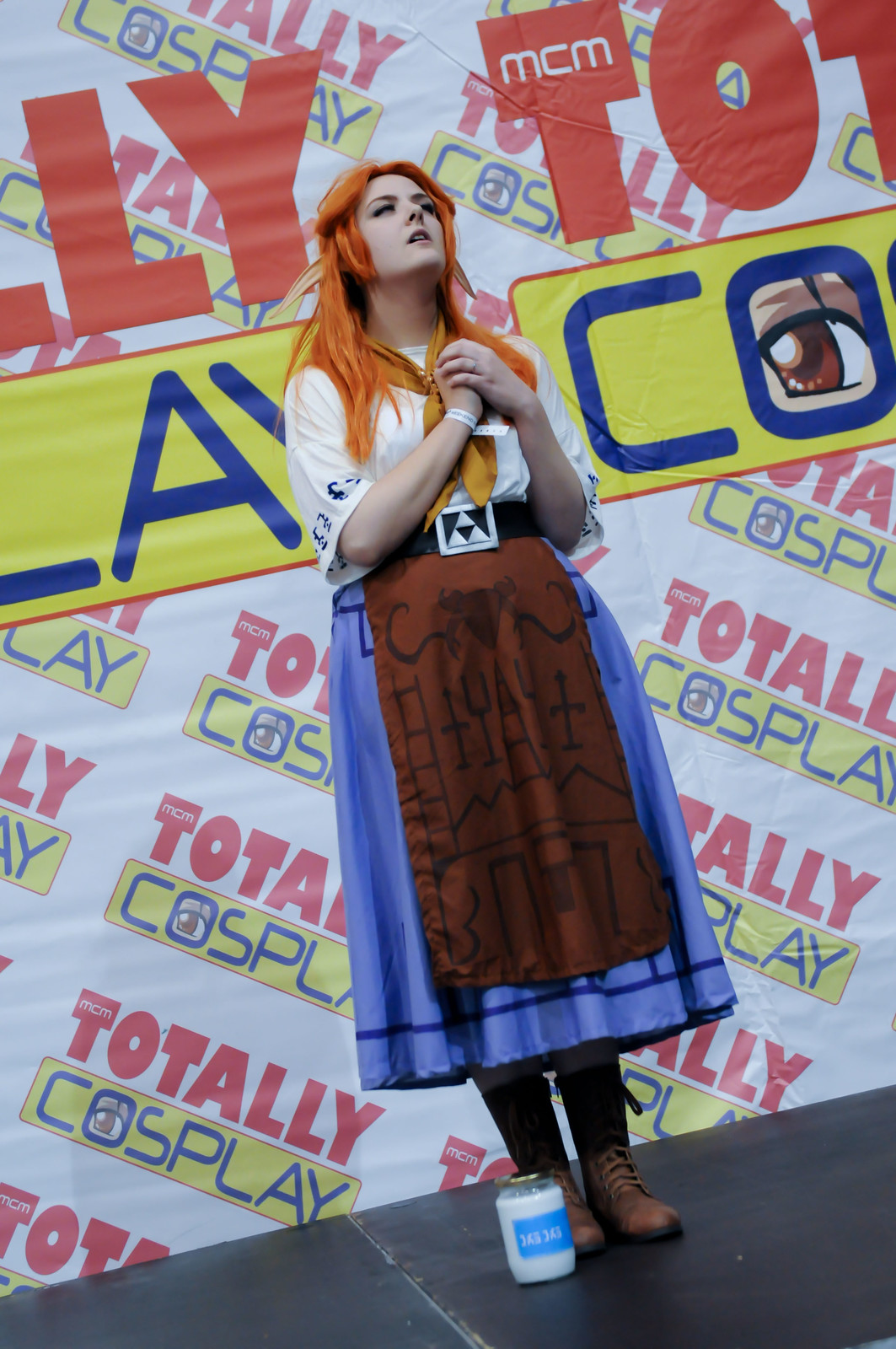In this photo, a young girl dressed in an elaborate costume stands in front of a "Totally Cosplay" banner, which features vibrant reds, yellows, and blues on a white background. She has striking dyed orange hair, possibly a wig, and wears a mustard-colored kerchief that complements her hair. Her light-skinned complexion is noticeable as she tilts her head slightly upward and to the left, eyes closed, with her hands clasped over her heart, evoking a prayer-like gesture. She's clad in a white top paired with a flowing bluish-purple skirt, a brown apron adorned with indistinct designs, and brown boots. Notably, she has a white wristband on. At her feet, there's a white container with a blue label, which might be for collecting donations. The ground below her is a dark gray slate color, adding contrast to her vibrant attire. The overall scene suggests she is embodying a character, perhaps performing or posing for a cosplay event.